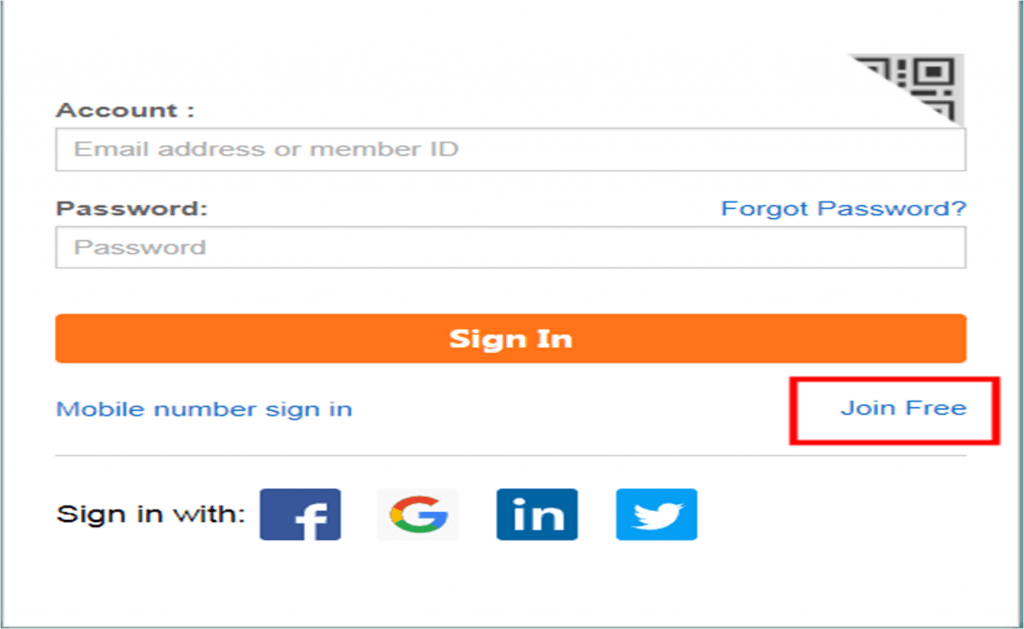The image depicts a login screen with a clean, organized layout. At the top right corner, there is a diagonally cut QR code with a gray background and black squares. Below the QR code is a text box labeled "Email address or member ID" in light gray font.

On the far left above this text box, the word "Account" is prominently displayed. Beneath the email text box is another text box for the user's password, with the label "Password" above it and "password" lightly printed inside the box as placeholder text.

Centrally located near the bottom of the middle section is a rectangular button with a bold orange background, containing the text "Sign In" in white, centered within the button and flanked by ample empty space on both sides. Below this button, to the far left, is the option "Mobile number sign in," and to the far right, the option "Join free."

At the very bottom, the image lists "Sign in with" followed by the logos of four social media platforms: Facebook, Google, LinkedIn, and Twitter.